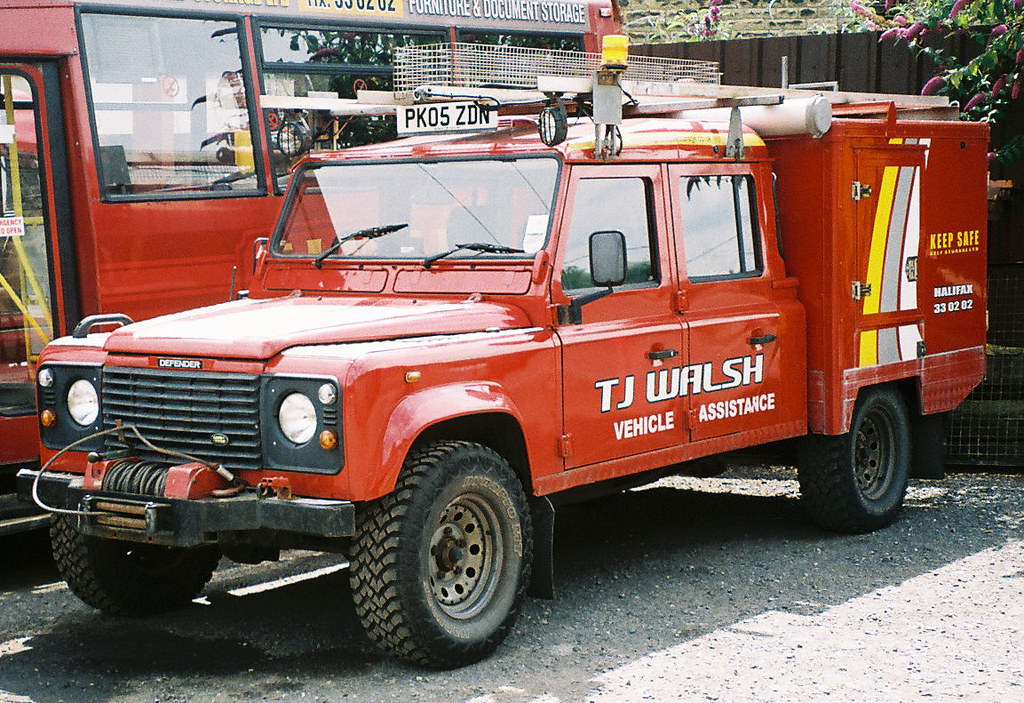This vibrant color photograph captures a red heavy-duty truck bathed in sunlight, parked on white gravel. The truck features a large cab with four doors and is equipped with heavy-duty treads. Instead of a standard truck bed, a sizeable boxy container with a small door is affixed to the back, indicating storage for tools or supplies. Affixed on top of the truck's roof is a rack loaded with various pipes, ladders, and additional equipment. The side doors bear white text that reads "TJ Walsh Vehicle Assistance," highlighting its purpose as an emergency or assistance vehicle. The front grill, black in color, showcases a sturdy red winch with a wire wrapped around it and a protruding cable, enhancing its rugged, utility-focused design. The vehicle's license plate reads PK05ZDN. Adjacent to this truck is a larger red vehicle, likely a bus, further emphasizing the setting in a gravel parking lot. The truck's robust and well-equipped appearance suggests its role in assisting and rescuing other vehicles from difficult situations.